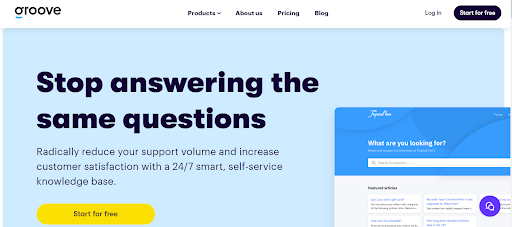The screenshot depicts a website titled "Groove," with its name prominently displayed in the upper left corner. Across the top navigation bar, from left to right, are the options: "Products" with a drop-down arrow, "About Us," "Pricing," and "Blog." On the upper right side, there is a "Login" option and a dark-colored tab with white text inviting users to "Start for Free."

The central area of the page features a light blue background with a prominent headline in large black text on the left side stating, "Stop Answering the Same Questions." Below this headline, in smaller, lighter-colored text, it reads, "Radically Reduce Your Support Volume and Increase Customer Satisfaction with a 24-7 Smart Self-Service Knowledge Base." Directly beneath this text is a yellow button that reads "Start for Free."

In the bottom right corner of the page, a segmented box is visible. The top part of this box is medium blue, while the bottom section has a lighter blue or light gray background. The text within this box is notably blurry and difficult to read, rendering most of it illegible. However, the legible part reads "What Are You Looking For?" followed by more unreadable text. Below this prompt is a rectangular search bar with a white background and a magnifying glass icon that invites users to "Search for Answers." Further down, there is more blurred text, with the second word appearing to be "Articles." Lastly, in the very bottom right corner, there is a circle with a blue-purple background, featuring an unidentified icon.